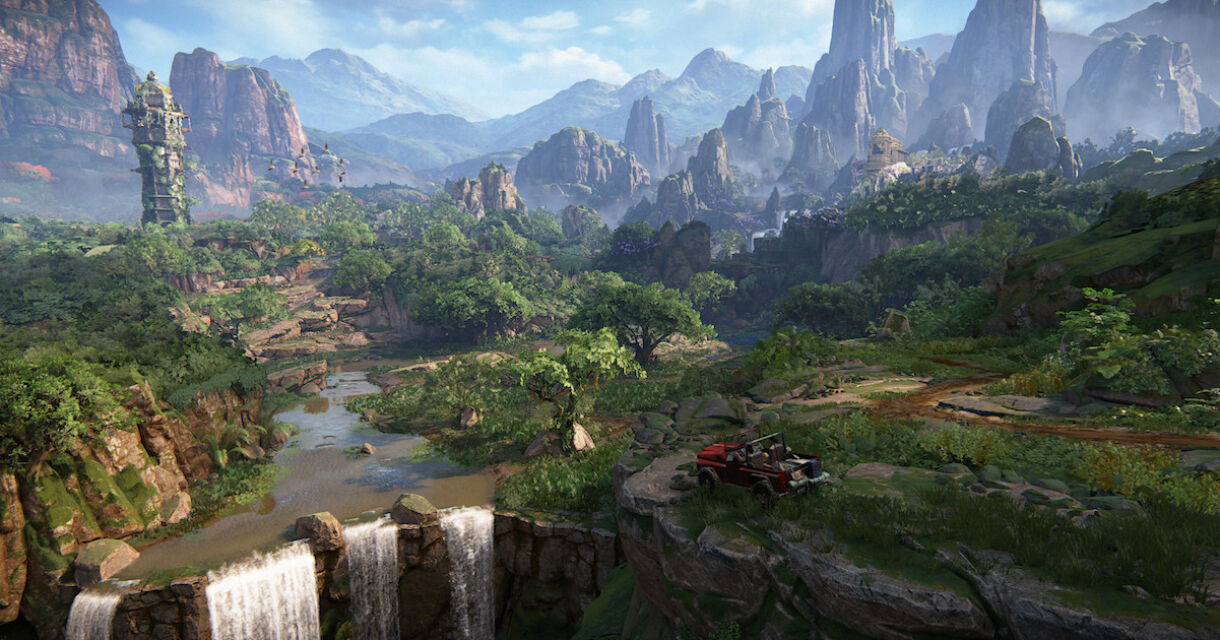This image is a detailed and serene depiction of a nature landscape, possibly generated by AI, with a blend of fantasy elements. In the background, there are numerous mountains with rock faces. The mountains start with brown hues in the foreground and transition to gray as they recede into the distance. Towering over this picturesque scene is a big blue sky adorned with white clouds, adding to the tranquility.

Lush green vegetation fills the landscape, with vibrant trees and grass carpeting the area. A rolling river meanders through the middle left of the scene, leading to four waterfalls cascading down between rocks at the bottom left, their white water contrasting with the greenery.

On the left side, a man-made rock tower covered in ivy and grass stands tall, resembling a lookout point. Toward the middle right, a red Jeep with its top down is parked precariously on a rocky cliff, with two people seated in the front seats, gazing over the scenic vista. This Jeep appears to be a focal point, symbolizing exploration and adventure amid the tranquil natural beauty.

The overall atmosphere of the image is both serene and majestic, blending the beauty of untouched nature with subtle hints of human presence.